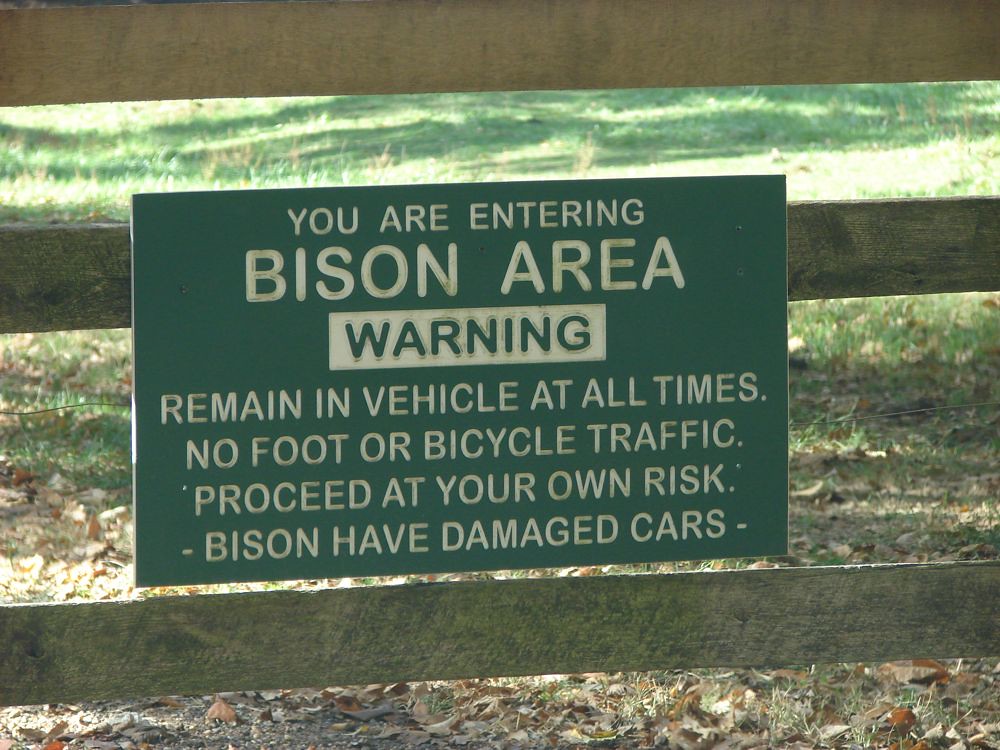This color photograph, taken outdoors during the daytime, features a wooden fence with three horizontal planks. Hanging slightly to the left on the middle plank is a green rectangular sign displaying a warning message in white letters. The sign reads: "You are entering bison area. Warning, remain in vehicle at all times. No foot or bicycle traffic. Proceed at your own risk. Bison have damaged cars." The word "Warning" is highlighted with a white background. In the foreground, the ground is scattered with brown leaves, suggesting fall, and brown grass, while behind the fence lies an expansive area covered with green grass. The fence itself is a brown-gray color, and the entire scene is bathed in sunlight, emphasizing the open and natural surroundings.